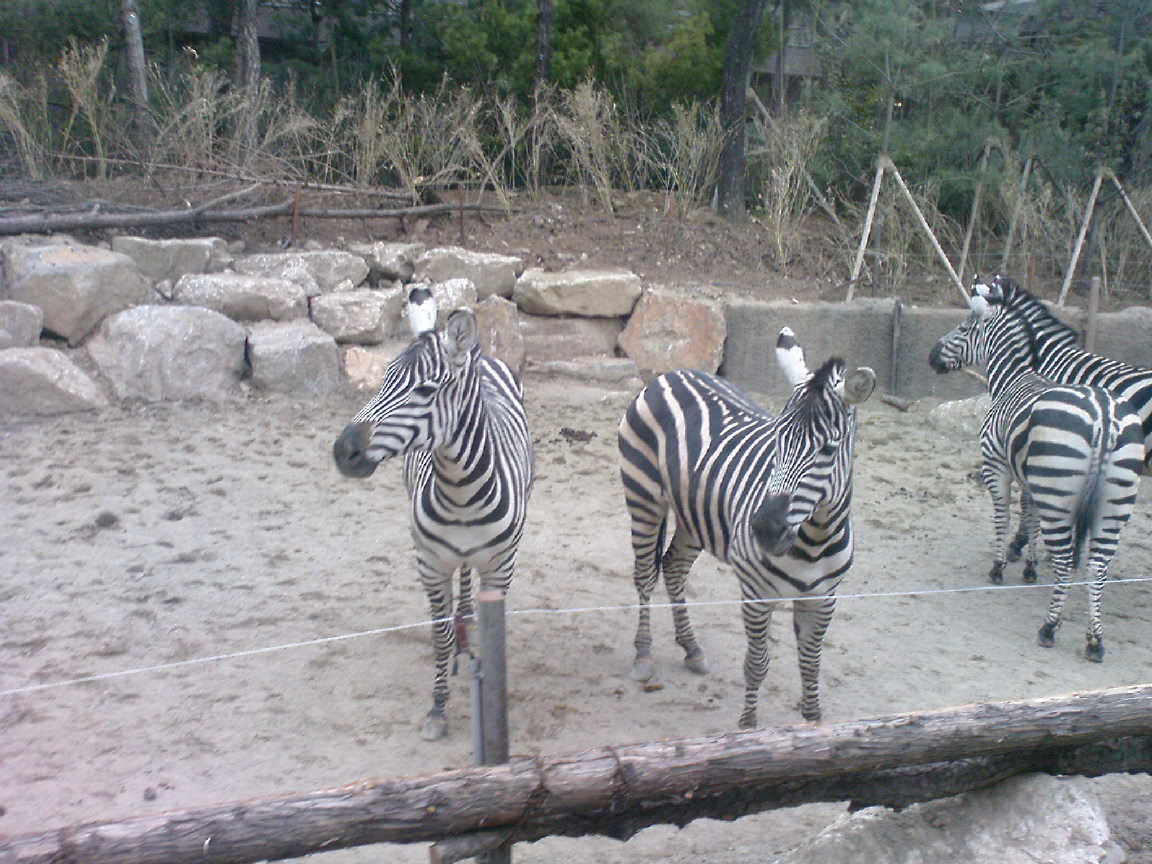This is a detailed photograph of a zoo enclosure housing four zebras. The setup includes a long, sandy ground where the zebras stand. In the foreground, the enclosure is secured by a wooden fence topped with an electrified wire. The zebras are positioned in a specific arrangement: two in the center face towards the camera, while the other two on the far right stand with their backs to us. Behind the zebras, the enclosure features a low stone wall or cement barrier, complemented with stacks of rocks. The backdrop rises with dense foliage, composed of bushes and tall trees, which is indicative of a natural, verdant environment. The general ambiance of the photograph is overcast, providing a muted lighting that subtly dims the scene without casting strong shadows.